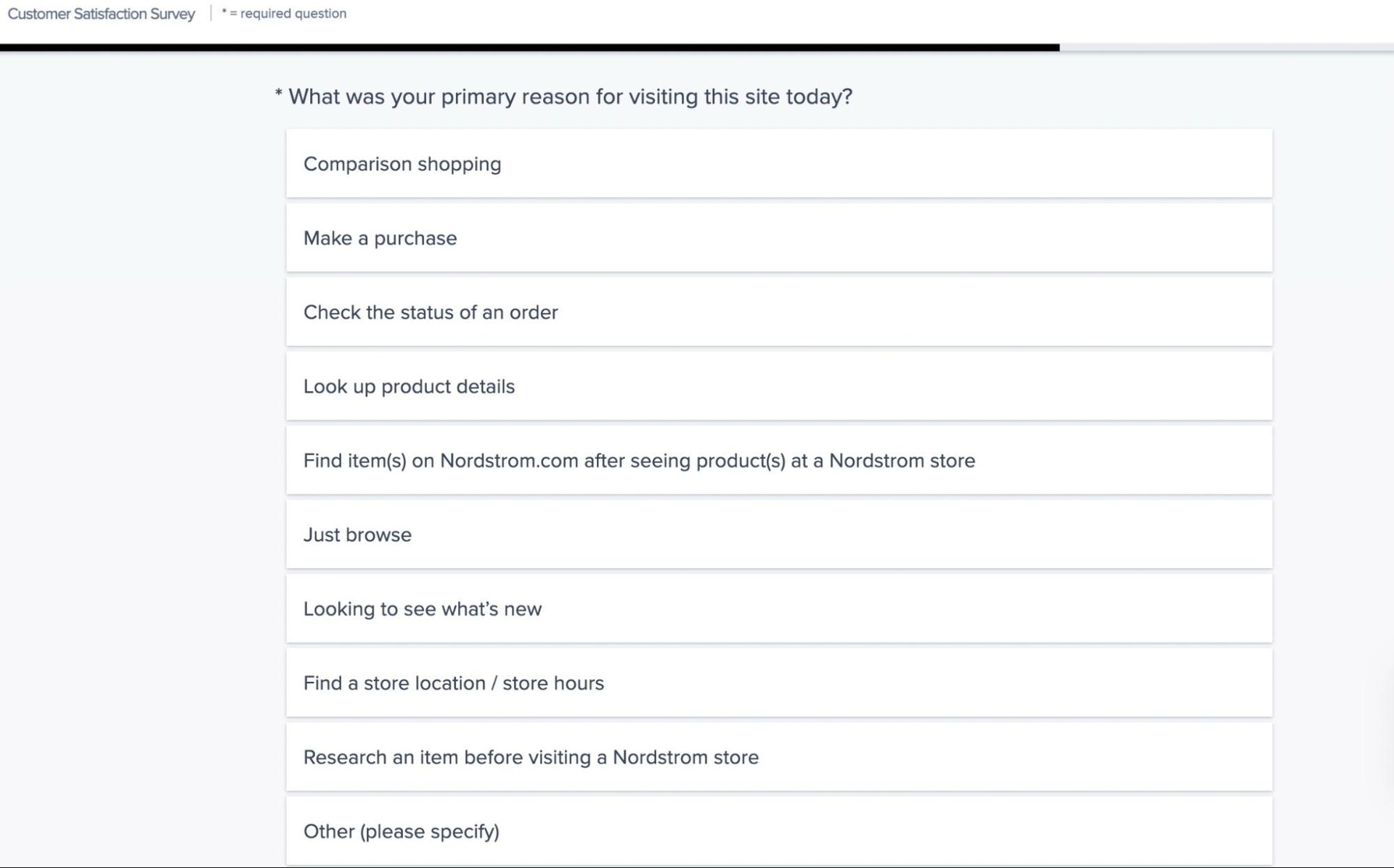The image showcases a webpage displaying a Customer Satisfaction Survey. In the top-left corner, the title "Customer Satisfaction Survey" is prominently displayed, followed by an asterisk and the note "* Required question," indicating the mandatory nature of the subsequent inquiries. Below, a black horizontal line spans the width of the section, providing visual separation.

Underneath the line, a bold prompt reads: "* What was your primary reason for visiting this site today?" followed by a list of possible responses, formatted as radio button options. The choices are:

1. Comparison shopping
2. Making a purchase
3. Check the status of an order
4. Look up product details
5. Find item(s) on Nordstrom.com after seeing product(s) at a Nordstrom store
6. Just browse
7. Looking to see what's new
8. Find a store location/store hours
9. Search an item before visiting

Each option appears clearly and concisely, helping respondents to easily identify and select their primary reason for visiting the Nordstrom website.